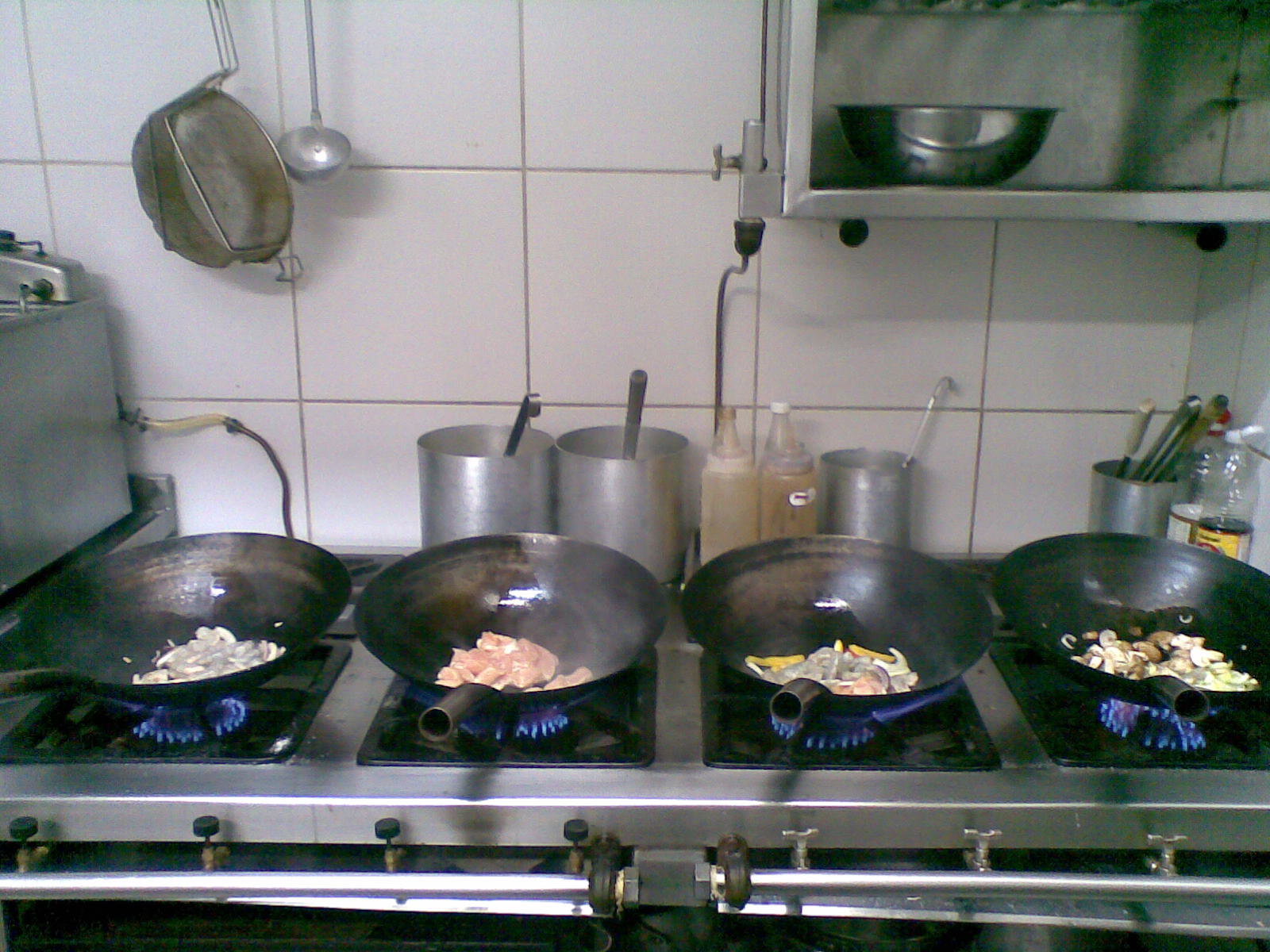The image depicts a bustling restaurant-style kitchen focused on a commercial gas stove with four large lit burners, each supporting a wok. The woks are filled with different food items: one appears to have mushrooms, another has pieces of chicken, a third seems to contain a mix of vegetables, possibly including peppers and onions, and the last wok also contains mushrooms. Behind the cooking area is a white tile wall, adorned with an array of stainless steel utensils, pots, strainers, and ladles hanging above. A stainless steel shelf situated above the stovetop holds a metal bowl, while the countertop is lined with aluminum containers filled with various cooking utensils. The scene suggests an active kitchen environment, likely in the midst of preparing a fresh order.